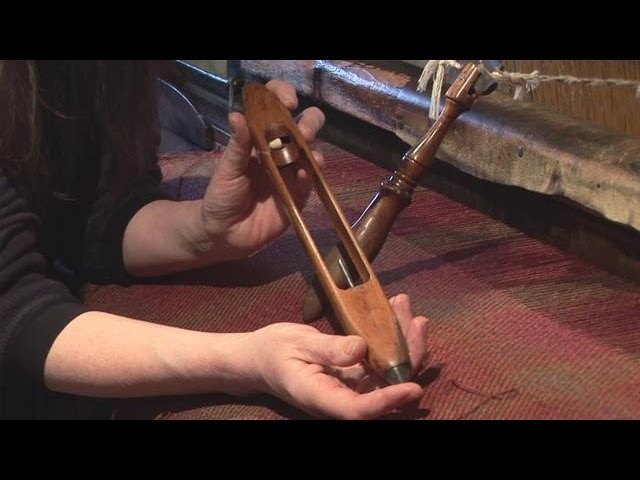In this color photograph, a white man with long brown hair and sleeves pushed up, positioned on the left side of the frame, is holding a wooden boat shuttle—a tool traditionally used for weaving fabric on a loom. He holds the shuttle vertically with one hand on the bottom and the other on the top, showcasing it in front of a historical wooden loom. The loom appears to be in use, as red fabric can be seen emerging from it at the bottom right of the image. The scene also includes a smaller wooden piece in the background, resembling a table leg, hanging from a cord. The backdrop features a flannel-patterned blanket in hues of red, pink, and brown, and a wooden wall or railing with a decorative cord draped across it, adding to the historical and rustic atmosphere of the photograph.